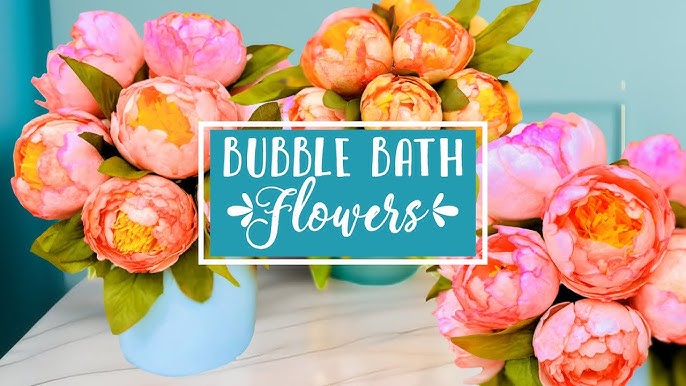The promotional image is rectangular, with the top and bottom sides twice as long as the left and right sides. At the center, a thin white line encloses a green rectangle, inside which white text reads "Bubble Bath Flowers." The background features three flower arrangements in cylindrical vases that are either light blue or dark green. The flowers have bulbous, spherical pink petals with yellow filaments in the center, green stems, and large green leaves. They are placed on a marble-like table surface with a blue-painted wall behind them.